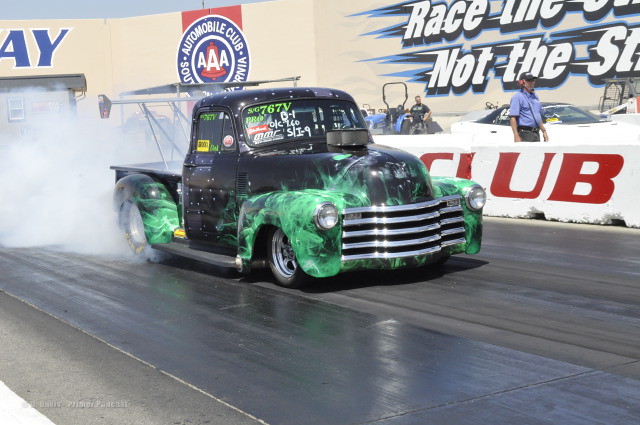A landscape-oriented image features a vintage 1950s-style black pickup truck, tricked out with lime green flames along the fenders, bumper, and wheel wells. The truck, fitted with a large spoiler and an exposed engine protruding from the front hood, is captured mid-motion on a slick, damp drag racing track, moving from the left side to the front right of the frame. Green, red, and white lettering, including "767V PRO D-1 S-I-9" and other unclear text, is seen on the truck's front windshield. Thick smoke billows from the rear tires, indicating intense acceleration. To the right of the truck, a low white concrete barrier with "Club" painted in red is visible, behind which stands a man in a pit crew headset. In the background, a blue tractor and another crew member can be seen near a white, Corvette-like car. A cream-colored wall adorned with advertisements, including partially legible phrases like "Automobile Club AAA" and "Race the," frames the scene.